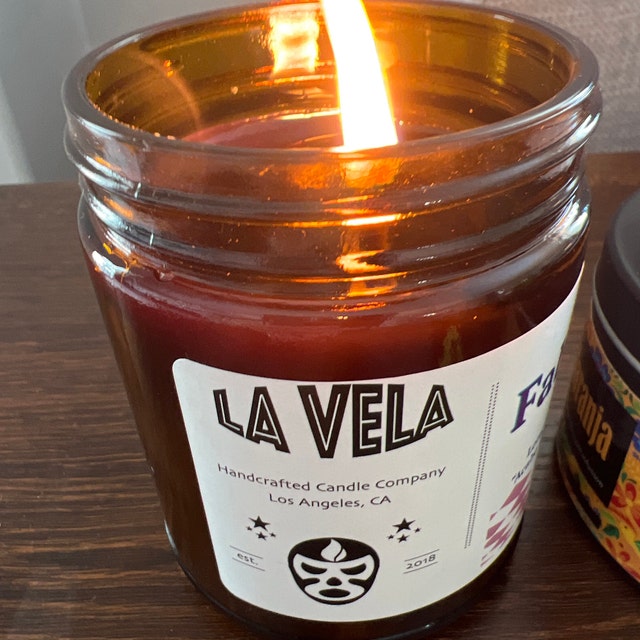This photograph features a lit candle placed centrally on a dark brown wooden table. The candle is encased in a cylindrical, clear glass jar with deep reddish wax inside. Prominently displayed on the white label of the jar is the brand name "La Vela" in black text, followed by the inscription "Handcrafted Candle Company, Los Angeles, California," also in black lettering. The label includes additional elements: a black and white Mexican luchador mask, two sets of four black stars, and the phrase "Established 2018" flanking the mask. A bright orange flame burns at the top of the candle. Positioned to the right of the candle is another round jar with a vibrant, multicolored label featuring yellow text that appears to read "Anja" within a black box, though the contents are unclear. The background shows a light gray wall occupying the top three-quarters of the image, reinforcing the serene and warm ambiance created by the illuminated candle.